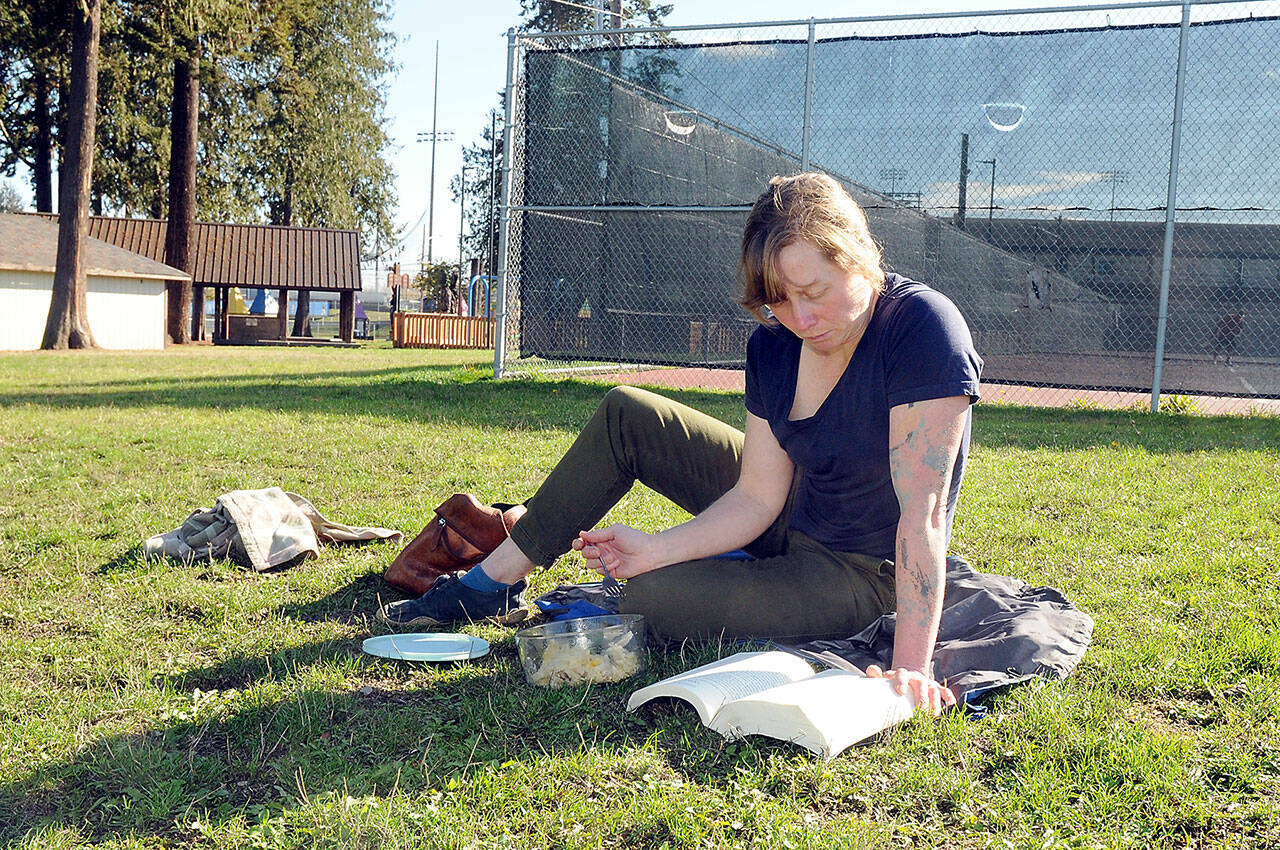In this photograph, a woman is enjoying a picnic in a park setting. She sits on a jacket spread on the grass, engrossed in reading a thick paperback novel or textbook. She is casually dressed in a blue t-shirt paired with army green pants, blue socks, and darker blue sneakers. Her brownish-auburn hair is tied back in a ponytail, revealing a tattoo on her left arm. The woman is eating from a glass container, the plastic lid of which lies beside her on the grass. Nearby, a brown purse rests by her foot, and further away, a piece of cloth or another item of fabric is on the ground.

The background reveals a diverse park environment with tall pine trees to the left. Behind the woman, there are tennis courts enclosed by a large chain-link fence and netting. Additionally, the scene includes a playground, a picnic shelter with tables, and a white building that might serve as restrooms or a small shed, all indicating a well-used public space. Utility poles and a small fence are also visible near the pavilion. The sun is shining brightly, adding a cheerful ambiance to the scene.